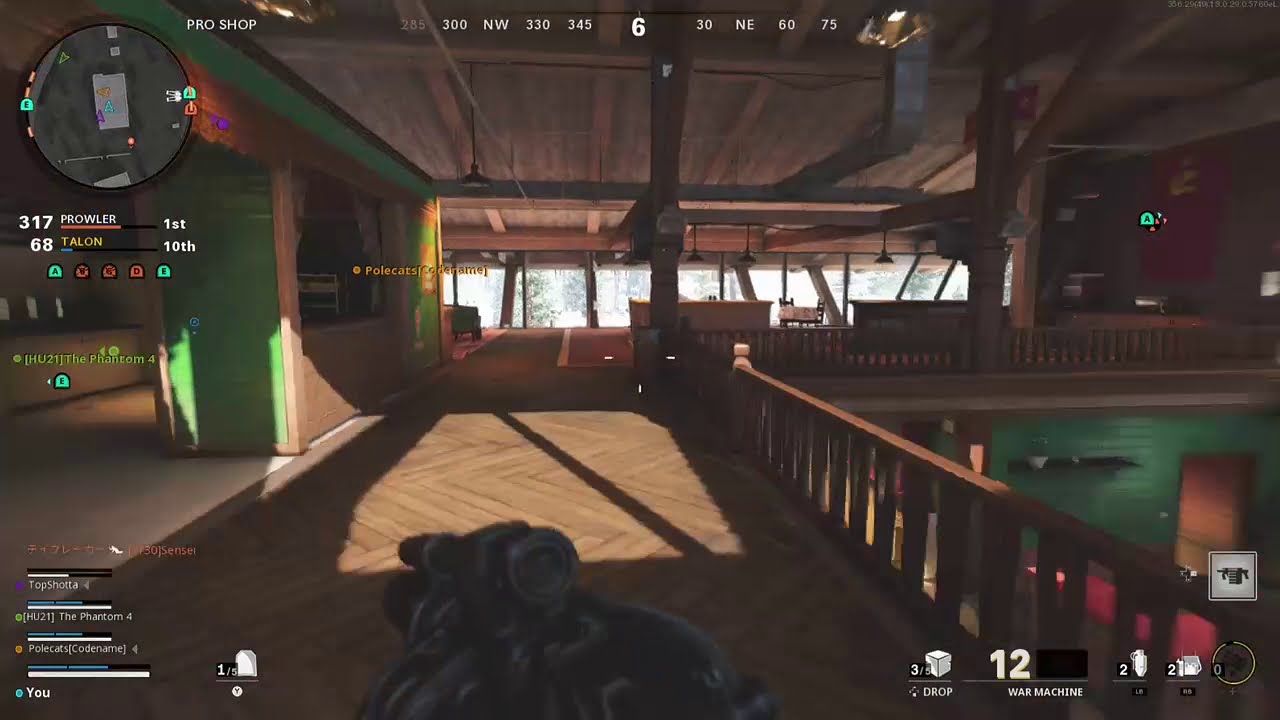This image is a detailed screenshot from a first-person point-of-view shooting game, possibly Call of Duty. The player is on the second floor of an indoor setting with wooden floors and green walls. The center bottom of the image prominently displays an animated assault rifle equipped with a scope. To the left of the screen, a compass shows directional information such as 317 Prowler, 1st, and 68 Talon, 10th, along with game control symbols labeled AXBDE. The lower left contains health bars and teammate names. On the right side, icons for a drop, a war machine, and accessible player-held objects are visible. The setting includes detailed interiors featuring a wooden ceiling, partial green-painted walls, a breakfast or service bar area, wood plank flooring, and railings. The top of the screen features directional degrees, ranging from 285 to 75, oriented northwest to northeast, with white numeric indicators such as 6 and 30. The color scheme predominantly consists of brown, white, and green.